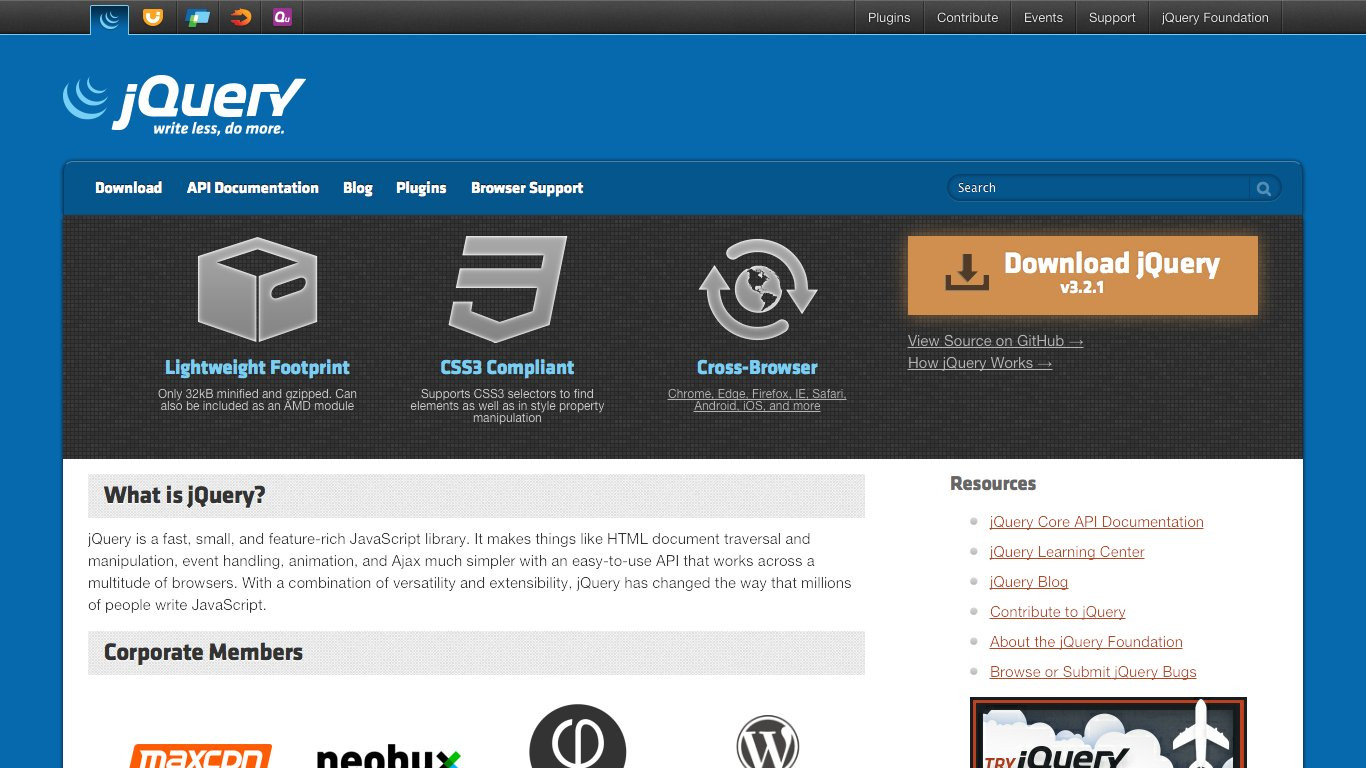The image depicts a computer screen displaying the jQuery website. The top section features a black banner adorned with colorful symbols on the left, representing blue, orange, green, red, and purple hues. To the right, the banner lists options like "Plugins," "Contribute," "Event Support," and "jQuery Foundation."

Beneath the black banner, the background transitions to blue, showcasing a blue wave symbol alongside the text "jQuery" in white, accompanied by the slogan "Write less, do more." Below this, a darker blue banner presents navigation options such as "Download," "API," "Automation," "Blog," "Plugins," and "Browser Support" in white text, with a search bar located on the right edge of this banner.

The subsequent section is divided into three informational boxes. The first box, gray in color, highlights "Lightweight Footprint" in blue. The second box features a backward E with a point at the bottom, signifying "CSS 3 Compliant." The third box shows a gray globe with two arrows encircling it and the phrase "Cross-Browser." Adjacent to these boxes, on the right, is an orange "Download Query" button accompanied by a download icon. Each of these boxes includes a brief description rendered in gray text.

Further down, the screen shifts to a white background with a gray banner titled "What is jQuery?" in black. This section contains a paragraph explaining the jQuery library. Below this, the segment titled "Corporate Members" appears, albeit with four logos of businesses that are cut off and not clearly visible.

In the lower corner, a "Resources" section is visible, listing six bullet points in orange text. At the bottom of this section, there's a call-to-action labeled "Try jQuery" alongside an airplane symbol, encouraging users to explore jQuery further.